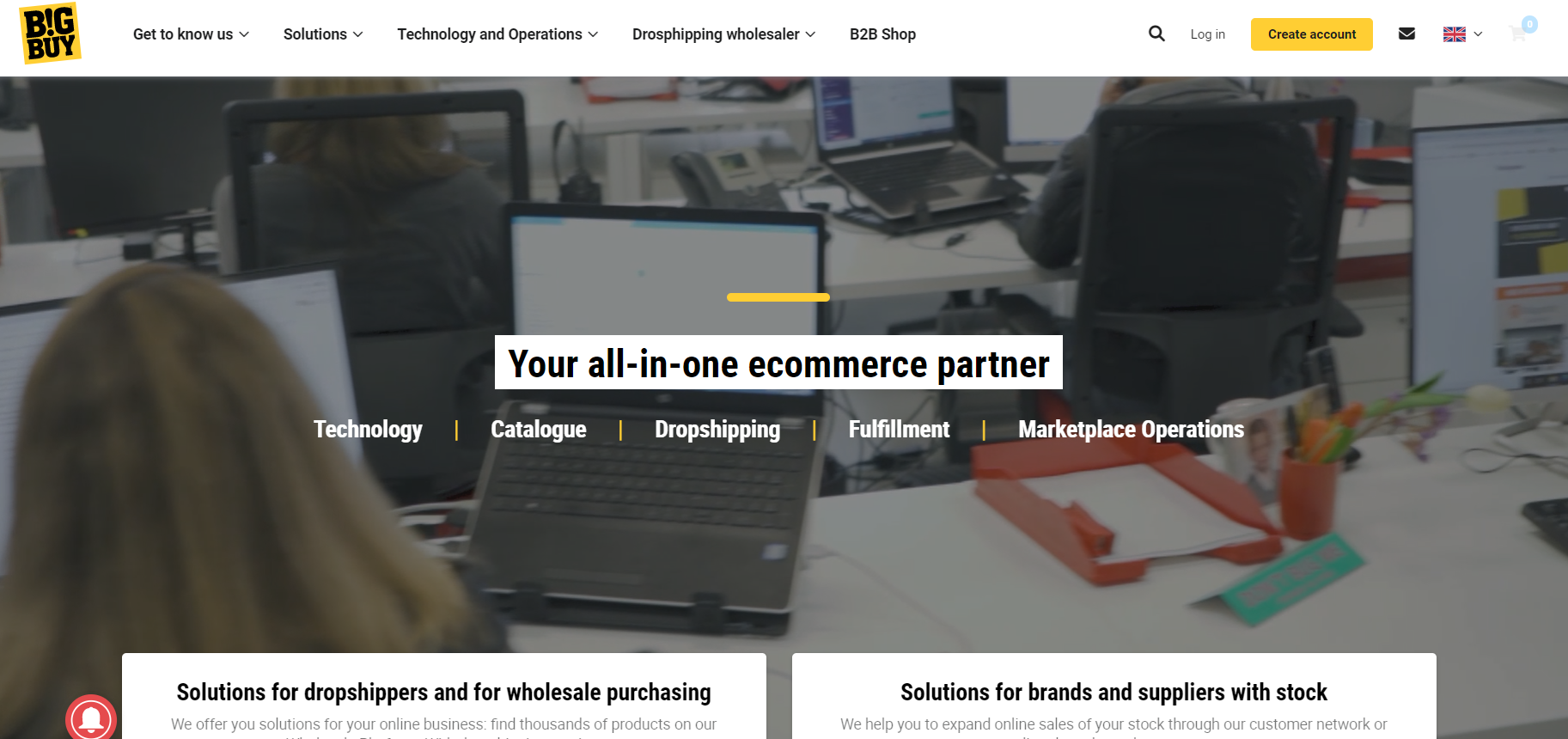Certainly! Here's a cleaned-up and detailed caption based on the provided description:

---

The homepage of Big Buy’s website features a sleek and user-friendly interface. At the top, the navigation menu includes several drop-down options: Get2KnowUs, Solutions, Technology, Operations, Dropship, Wholesaler, and B2B Shop. To the right of the menu, there are icons for search, login, create account, and mail (represented by an envelope). Additionally, there is a British flag icon for language selection and a shopping cart icon, indicating it contains one item, though the number is faint.

Central to the page is a professional photograph of an office environment underscored by the tagline, "Your All-in-One eCommerce Partner." Beneath this, various service categories are highlighted: Technology, Catalog, Dropshipping, Fulfillment, Marketplace Options, and Operations, specifically tailored for Dropshippers and Wholesale Purchasing.

The page emphasizes Big Buy’s comprehensive offerings for online businesses, boasting thousands of products available, although part of the text is cut off. It also mentions solutions for brands and suppliers to expand their online sales through Big Buy’s customer network.

The website’s color palette includes shades of yellow, white, black, red, blue, green, gray, and brown, creating a visually rich and appealing interface designed to support and enhance the experience of dropshippers and eCommerce businesses.